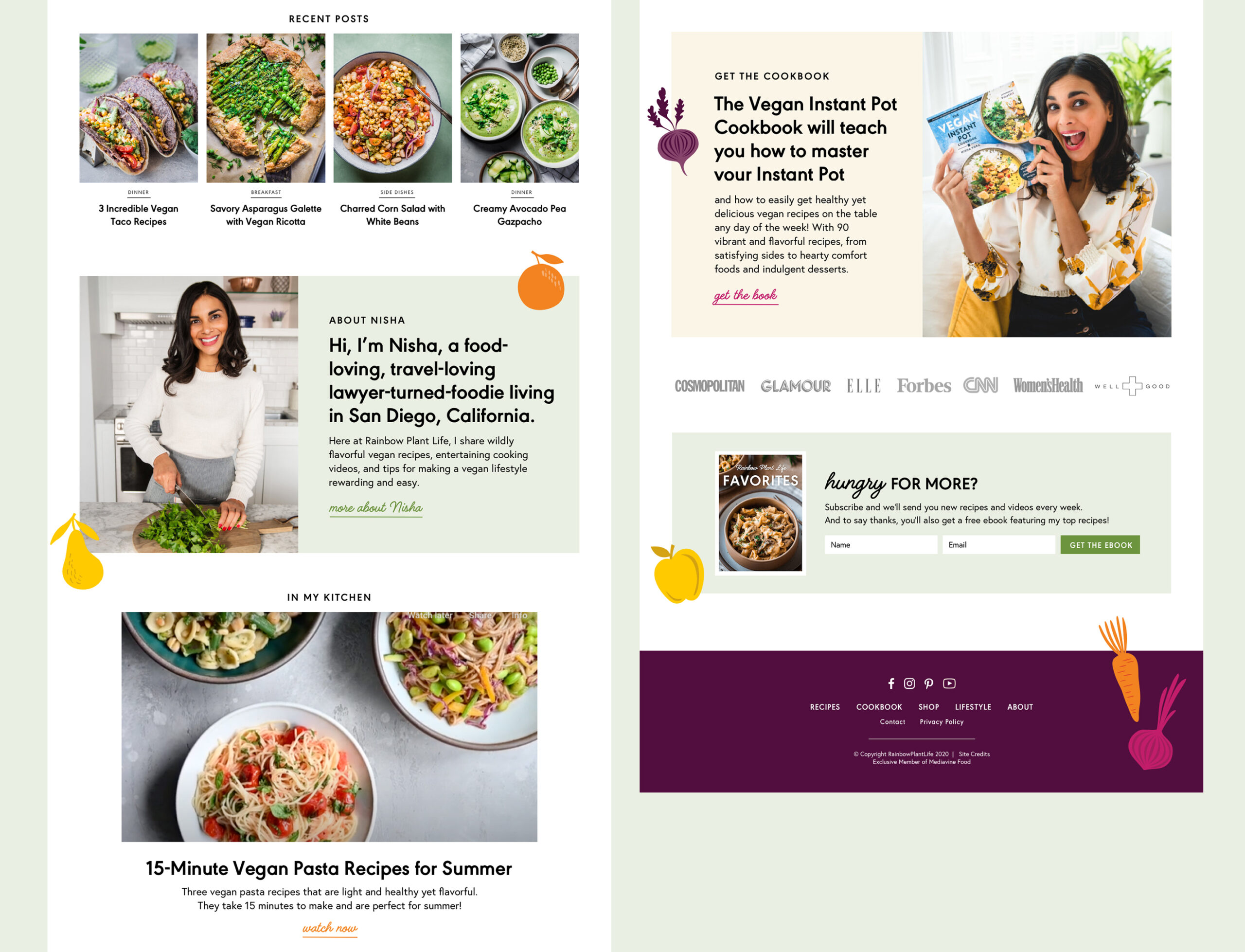This is an image of a vibrant cooking website dedicated to Nisha, a lawyer turned food enthusiast residing in San Diego, California. The website features a dual-pane layout with recent blog posts prominently displayed on the left. Nisha's blog showcases her passion for food and travel, emphasizing quick and easy recipes such as a "15-minute Vegan Pasta Recipe for Summer." 

At the top of the site, there are multiple categories highlighting different recipes, including unique dishes like "Charred Corn with Beans." Nisha appears to publish daily recipes, offering inspiration for everyday cooking.

Additionally, she has authored a "Vegan Instant Pot Cookbook," which aims to help readers master the use of their Instant Pot. A section labeled "Hungry for More" prompts visitors to sign up for updates, ensuring they never miss a new recipe or post. 

Near the bottom of the page, there is another clickable option for further exploring her website. This section also notes Nisha's media appearances in prominent publications and networks such as Cosmopolitan, Glamour, Forbes, and CNN, indicating her recognition and credibility in the culinary world.